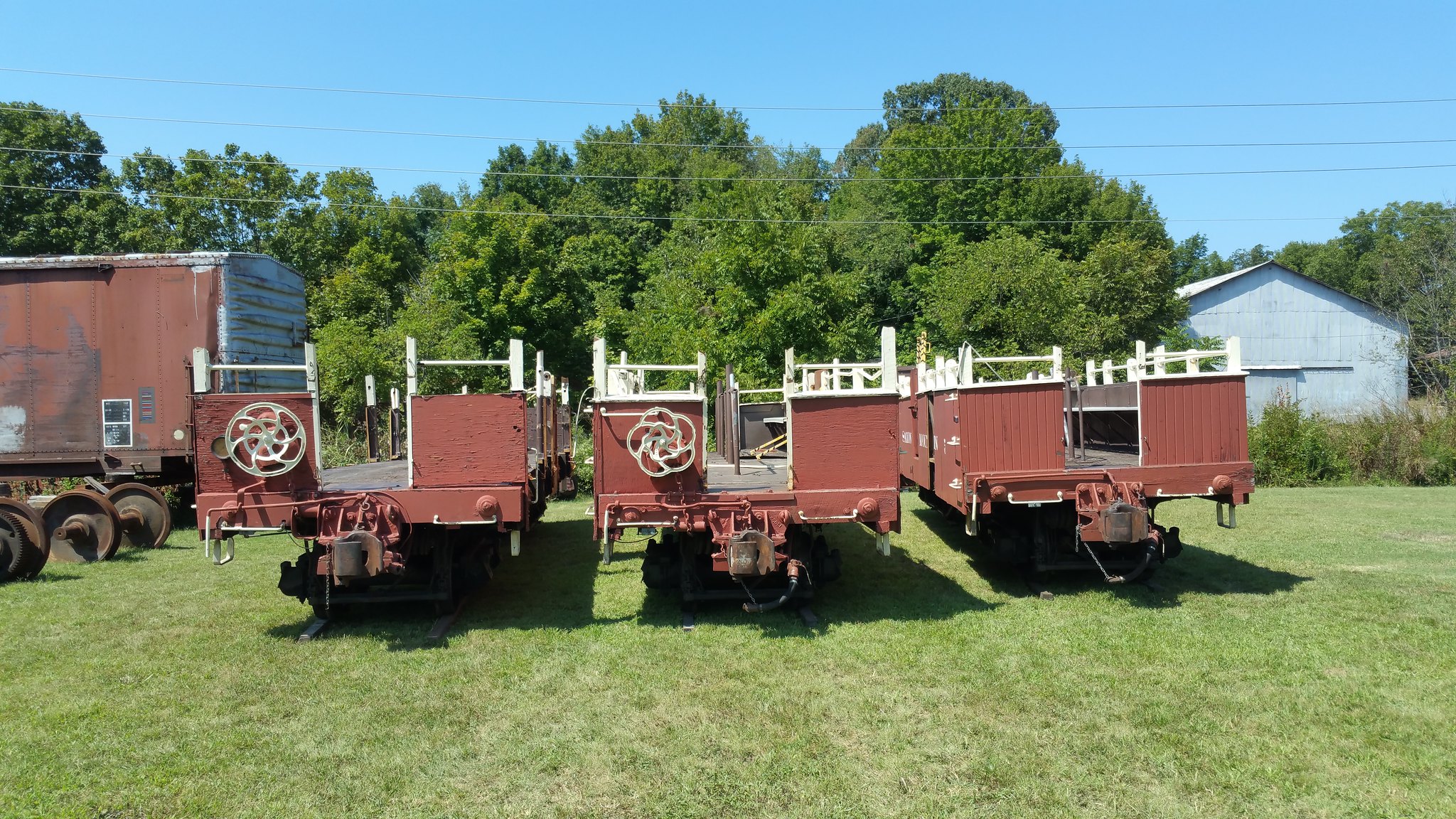This photograph captures a serene outdoor scene on a well-maintained property, characterized by a lush green field and a backdrop of tall, leafy green trees, likely oaks. The sky overhead is a brilliant blue, further enhancing the picturesque quality of the setting. Prominently featured in the foreground are three sizable maroon-colored trailers, each equipped with a hitch at the front. These open-bottom trailers are adorned with decorative white designs, resembling flowers and fan blades, on their sides. Two of the trailers notably have white bar railings along their edges.

The trailers, likely intended for carrying goods or people—possibly for hayrides—suggest usage of a powerful vehicle, such as a truck or tractor, to tow them. The neatly cut grass beneath them and the black wheels further signify their readiness for transit. To the right, partially visible, is a white building resembling a barn, with a touch of its roof showing. Additional structures in the background include an old, elevated maroon train car and a red building, hinting at the property being a farm. Power lines can be seen running across the tree line, completing the composition of this rural landscape.